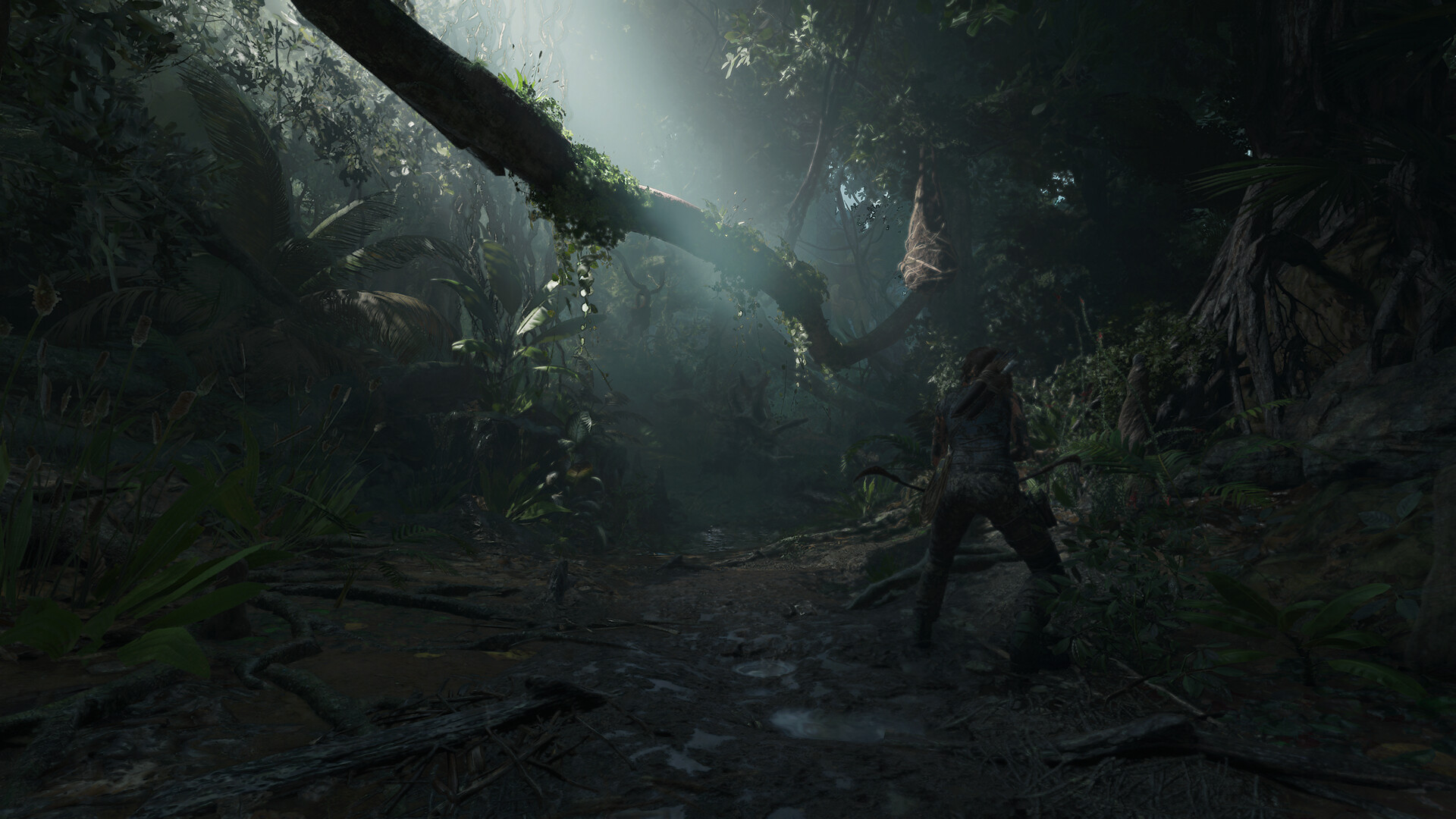In this detailed image from a video game, a dense jungle setting is illuminated by light filtering in from the canopy above. Dominating the upper middle section of the scene, a large tree branch extends from the top left, draped with greenish vines. The forest floor below is muddy, strewn with foliage, dead sticks, and various weeds. To the right, tropical vegetation thickens, alongside a tree entwined with dead vines. In the center-right of the image stands a woman, identified as Lara Croft from the 2012 remake of Tomb Raider. She is depicted in camouflage jeans, with long brown hair tied in a ponytail. Lara is armed with a short bow aimed toward the ground, and she carries two quivers on her back. Additional gear includes a canteen and a survival knife. Despite the camouflaged outfit, her vigilant stance and the bow partially hidden by her body mark her readiness. Lara appears to be looking upwards towards the canopy, possibly scouting the terrain.